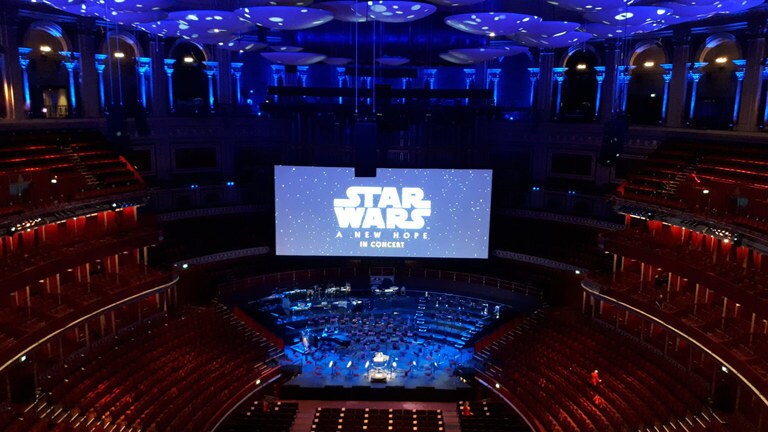The image depicts a grand, circular amphitheater-style concert hall with three tiers of red seats, which are largely empty. The photograph, taken from an elevated vantage point, looks down upon a stage set up for an orchestral performance. In the center of the scene, a massive projected screen displays "Star Wars: A New Hope in Concert" in white text against a light blue background. Below the screen, music stands are arranged, awaiting the orchestra. The ambient lighting creates a dramatic atmosphere: blue lights ring the upper perimeter of the room, casting a blue hue over the orchestra area, while white lights illuminate the red seats. The ceiling features unique, upside-down mushroom-like structures adorned with blue lighting, enhancing the theatrical feel. On the floor, a man in a red jacket and a woman beside him are the only visible attendees. The theater's design includes curved rows of seating extending up the left and right sides, with private viewing booths higher up, separated by walls and lit by arches and pillars, adding to the architectural grandeur.